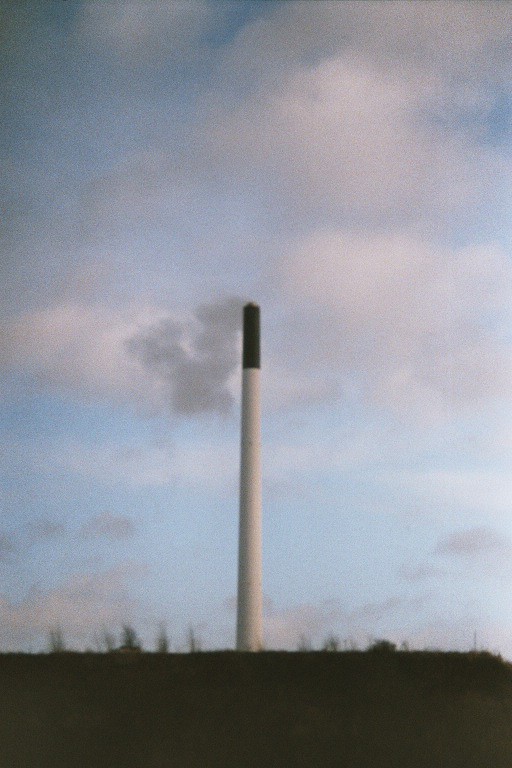The image features a tall, white smokestack standing prominently in the center, extending from near the bottom to the upper two-thirds of the frame. The base of the smokestack is surrounded by a blurry, brown ground with patches of dark vegetation and weeds. The top of the smokestack is marked by a darker, mostly black section from which gray smoke is billowing out and dispersing into the sky. The sky, which takes up the majority of the image, is an expanse of vivid blue interspersed with scattered, gray clouds. In the distant background, you can see tree branches peeking up from the horizon. Despite the photo's fuzzy quality and old appearance, it captures a daytime scene, possibly taken in the evening.